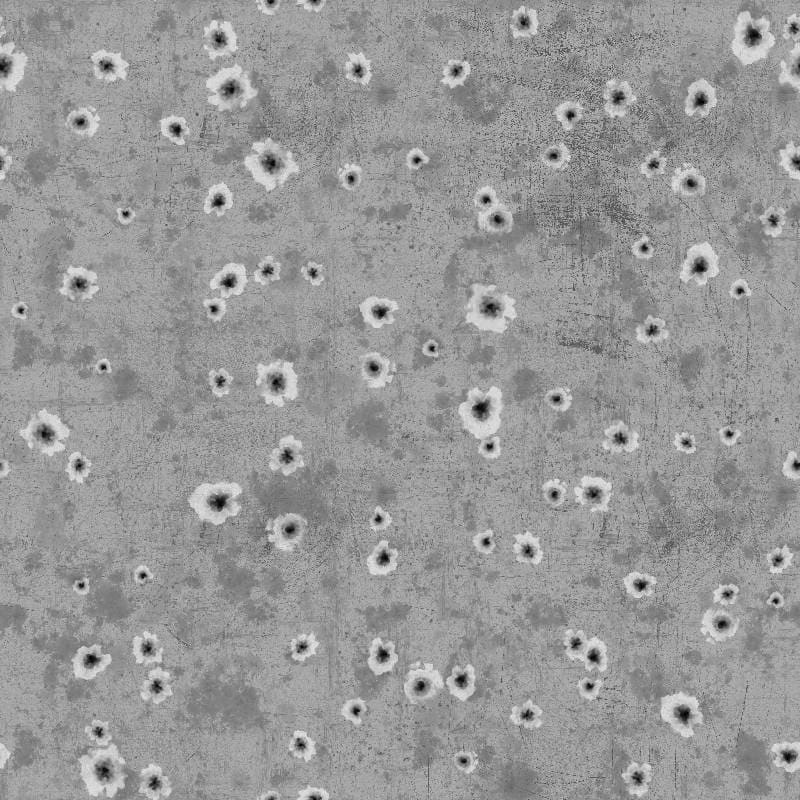This black-and-white image appears to be taken from a microscope, capturing an intricate, detailed view of an unidentified material or structure. The background features a light gray hue, sporadically patterned with dark gray patches and random crosshatched black lines reminiscent of scratches. Dominating the composition are numerous circular structures scattered uniformly across the entire image, each resembling a flower with its intricate layers. At the core of each structure lies a pronounced black center, encircled by a gray ring, which is then surrounded by a large, diffuse white area. These flower-like formations, though not actual flowers, proliferate throughout the visual field, adding to the image’s complexity and intrigue, suggesting a highly magnified, microscopic world.